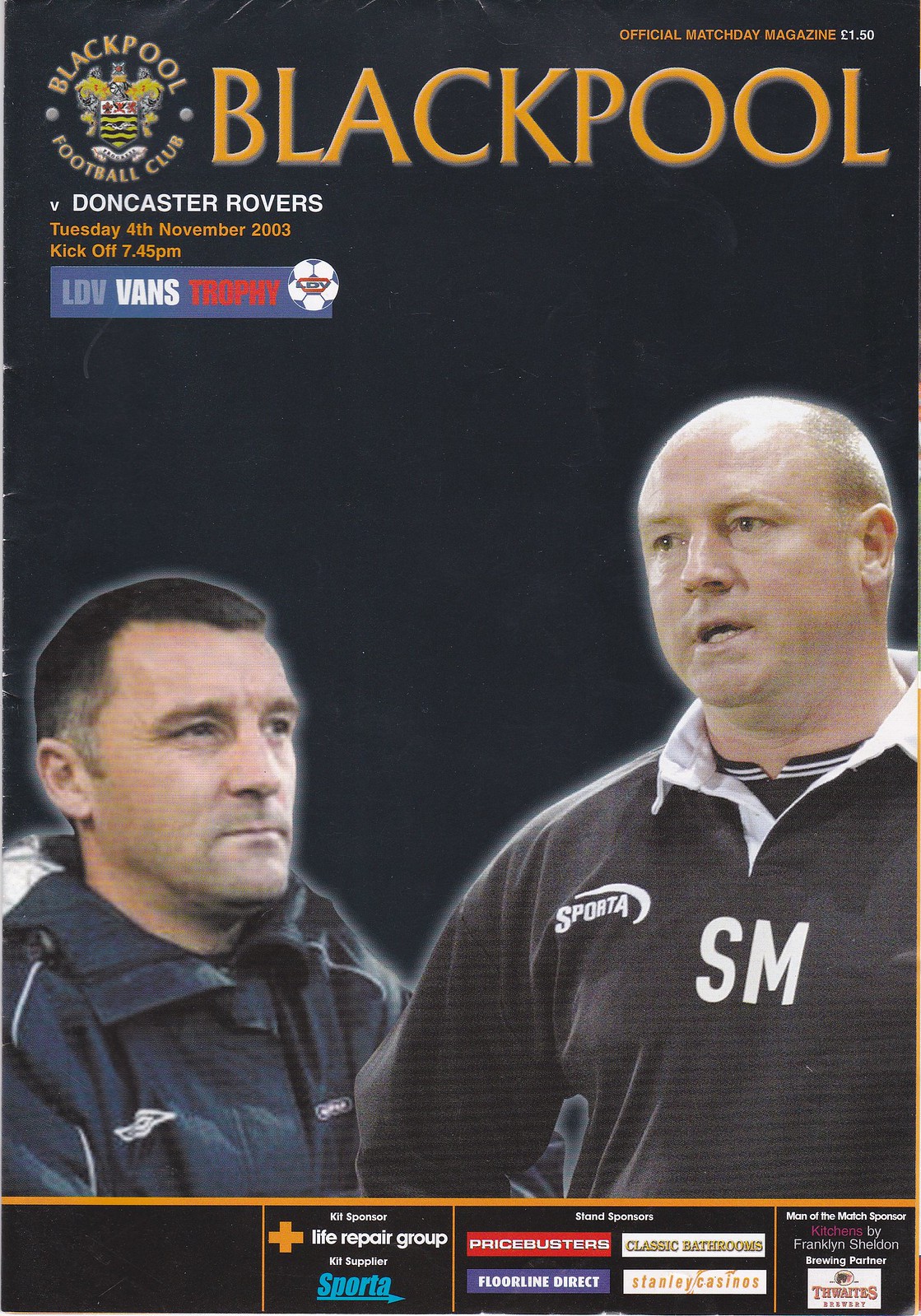The image is the cover of an official match day magazine for a European football club, specifically Blackpool FC versus Doncaster Rovers on Tuesday, 4th November 2003, with a kickoff at 7:45 p.m. The magazine, priced at £1.50, features a predominantly black background. In the upper left corner, the Blackpool Football Club's coat of arms is displayed, depicting two lions facing opposite each other with a shield that has three red stars on top. Next to the coat of arms, in golden text, it reads: "Official Match Day Magazine £1.50." Below, in white and gold text, details of the match are provided. A banner labeled "LDV Vans Trophy" appears beneath the match details, with a blue and white soccer ball next to it.

The cover prominently features two men against a black backdrop. On the left, a Caucasian man with short, cropped dark hair and a touch of white around his ears, wears a black coat and looks to the right. This figure is seen from mid-chest up. On the right, a bald Caucasian man with light-colored hair at the back of his head, dressed in a long-sleeved black shirt with a white collar and the initials "SM" in Sporta on the front, looks left; this man is visible from the solar plexus up. A thin gold pinstripe separates the image of the men from the bottom segment of the magazine cover, which lists several sponsors. These include "Kit Sponsor: Life Repair Group," "Kit Supply: Sporta," "Stand Sponsors: Price Busters, Floor Line Direct, Classic Bathrooms, Stanley Casinos," "Man of the Match Sponsor: Kitchens by Franklin Sheldon," and "Brewing Partner: Thwaites Brewery."